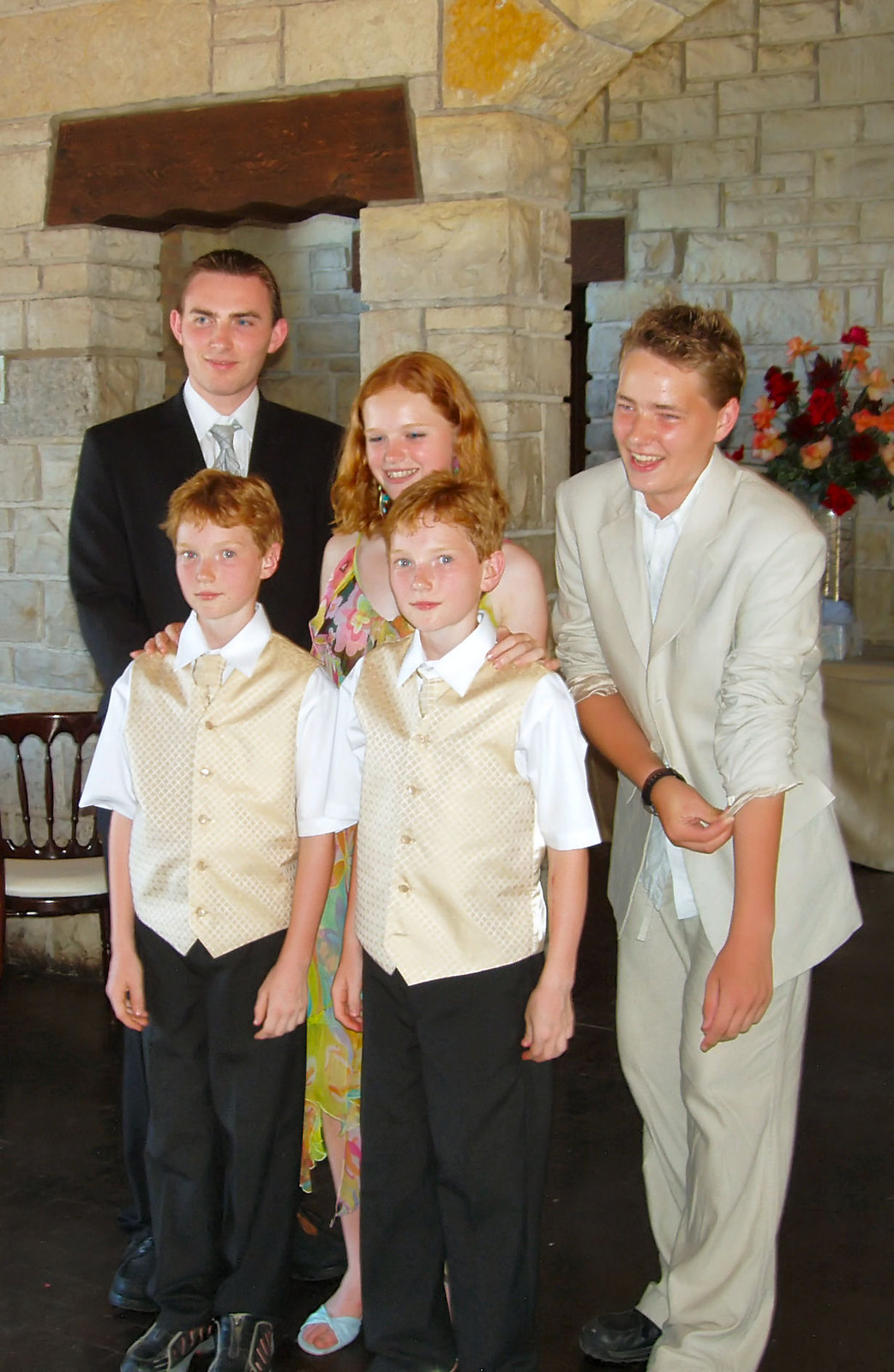This photograph shows a group of five young people, likely family members, gathered inside a stone-walled church. In the front are two identical twin boys with short red hair and blue eyes, dressed in champagne-colored button-up vests over white short-sleeved shirts, beige or golden ties, and black slacks. They are smiling slightly and looking at the camera. Behind them stand three older youths. On the left is a tall young man wearing a black suit, white shirt, and silver tie. In the middle, a girl with wavy red hair, adorned in a floral spaghetti strap dress with blue earrings, is smiling with her hands resting on the shoulders of the twin boys in front of her. To her left is another young man, taller than her but shorter than the boy in black, wearing a slightly oversized beige suit with a white shirt, his sleeves rolled up to his elbows, and smiling at the camera. The background features stone columns, walls, and a table with a cloth and a vase of multicolored fake flowers, suggestive of a formal event, possibly a family function, wedding, or first communion.